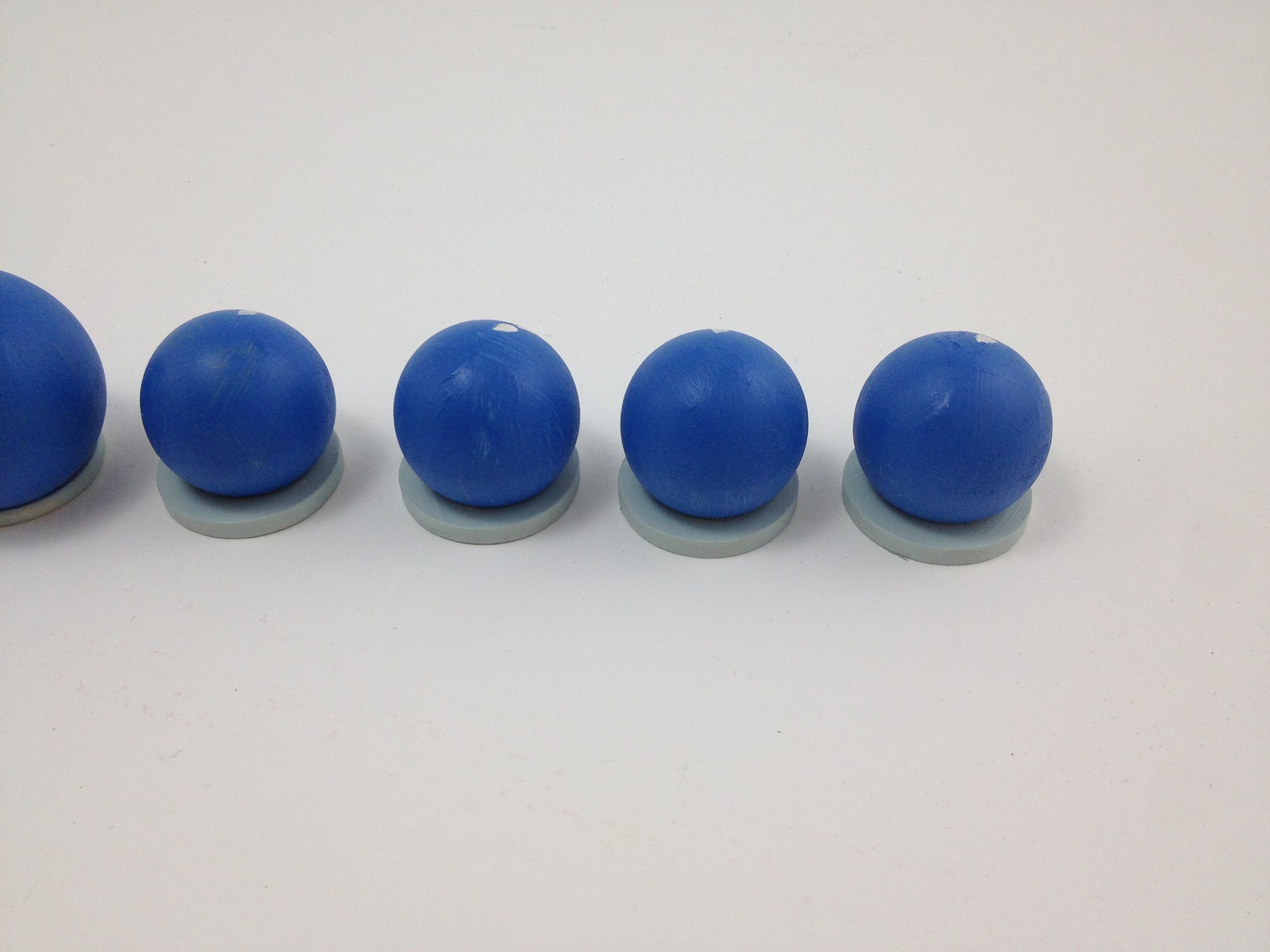This indoor color photograph features five identical dark blue balls, each mounted on gray circular bases, arranged in a horizontal row on a white background. The image is taken from a slightly elevated angle, looking down at the surface to the right. The balls, each about two inches in diameter, are evenly spaced, with the leftmost ball only partially visible and slightly larger than the others. The balls have chipped paint, revealing their underlying material, which gives them a worn, rubbery appearance. The soft, even lighting eliminates any shadows, presenting a clear view of the scene. There is no text or any other markings in the image.